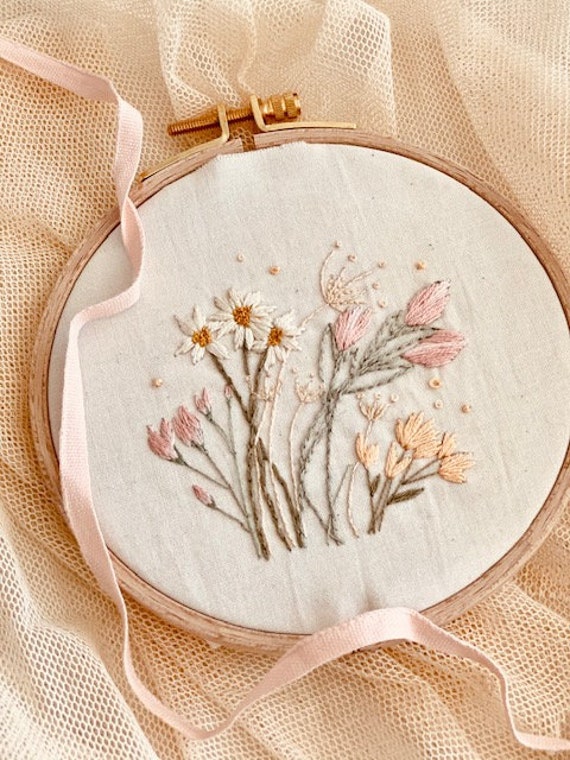The image portrays a meticulously crafted embroidery piece set within a wooden circular frame, secured at the top by a gold screw nut. This delicate artwork features a flax-colored linen fabric adorned with a complex bouquet of various three-dimensional flowers made from thread. The vibrant floral arrangement includes white-petaled daisies with golden-orange centers, clusters resembling Queen Anne's lace, as well as myriad other flowers in shades of pink, peach, and yellow. Beneath the embroidery hoop, the background consists of a soft, light pink mesh fabric, enhancing the visual appeal. A peach-colored ribbon elegantly meanders around the hoop, originating from the top left corner and gracefully trailing off at the bottom right. The professional quality photograph is perfectly lit and sharply focused, showcasing the intricate details of the handiwork, suggesting it could be a piece found on a high-end craft blog or used to adorn a tasteful home setting.